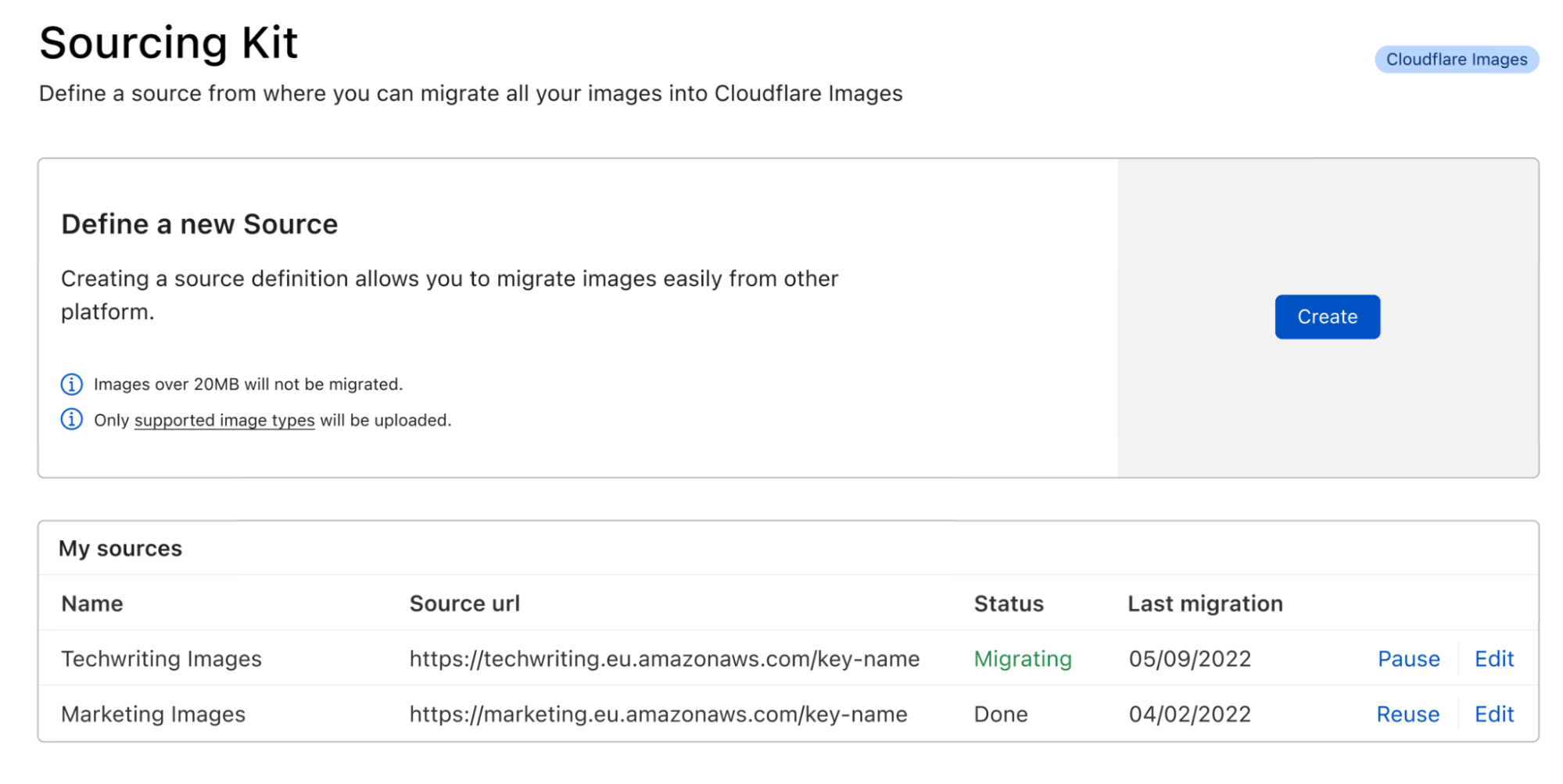**Detailed Caption for Cloudflare Image Migration Interface**

The interface has a clean design with a white background and mostly black text. In the top-left corner, "Sourcing Kit" is prominently displayed in bold, large font. Below this, in smaller text approximately half the size, it reads: "Define a source from where you can migrate all your images into Cloudflare Images."

In the top-right corner, "Cloudflare Images" is written in blue. Below this, there's a substantial horizontal box labeled "Define a New Source." This box includes the text: "Creating a source definition allows you to migrate images easily from one platform to another." Additionally, there is an information icon (denoted as an eye within a circle) stating, "Images over 20 megabytes will not be migrated. Only supported image types will be uploaded," with the phrase "supported image types" underlined. To the right of this descriptive box, a blue "Create" button is displayed.

Below this section, there is a secondary box titled "My Sources" which is the second of two distinct sections. This section consists of four columns labeled: Name, Source URL, Status, and Last Migration. Under the "Name" column, the first entry is "techwritingimages" (written as one word). The corresponding Source URL is "techwriting.eu.amazonaws.com/key-name". The status is indicated by a green label stating "migrating" with the date "5-9-2022." Options to "Pause" or "Edit" are available in blue text.

The second entry under the "Name" column is "marketingimages." The Source URL is simply "marketingEU." The status for this entry is marked as "done" on "4-2" with the note "migrated." There are also options to "Reuse" or "Edit" next to this entry, indicated by blue text.

The overall interface is designed to facilitate the easy migration of images from different sources to Cloudflare Images, emphasizing clarity and usability with important functions and statuses easily accessible.